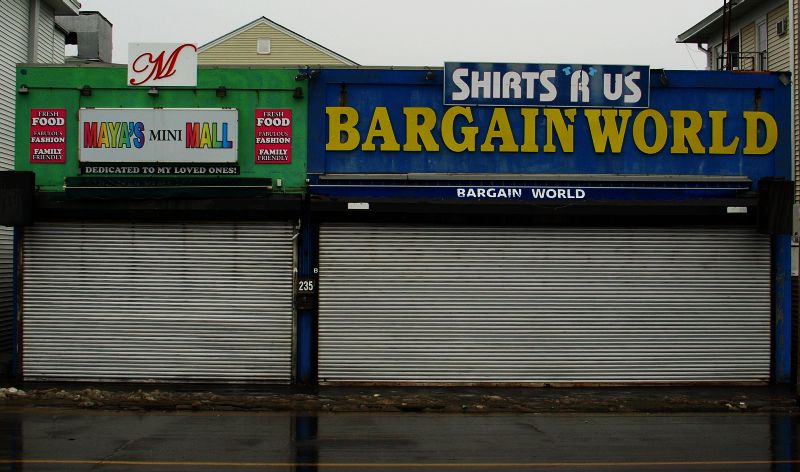Captured in this photograph is a pair of small businesses with their metal shutters rolled down to the ground, clearly indicating that they are currently closed. The establishment on the left, with its green facade, is named "Maya's Mini Mall," and bears the heartfelt dedication "Dedicated to my loved ones." The signage below proclaims offerings of "Food, Fashion, and Family," although the final words are too minute to decipher. The adjacent business on the right, slightly larger and sporting a blue exterior, is called "Shirts R Us," with the tagline "Bargain World" displayed beneath. The backdrop of the photograph reveals a white, cloudy sky and surrounding buildings that resemble residential apartments, giving the scene a cozy, tucked-away feeling, as if these businesses are nestled between two apartment complexes.